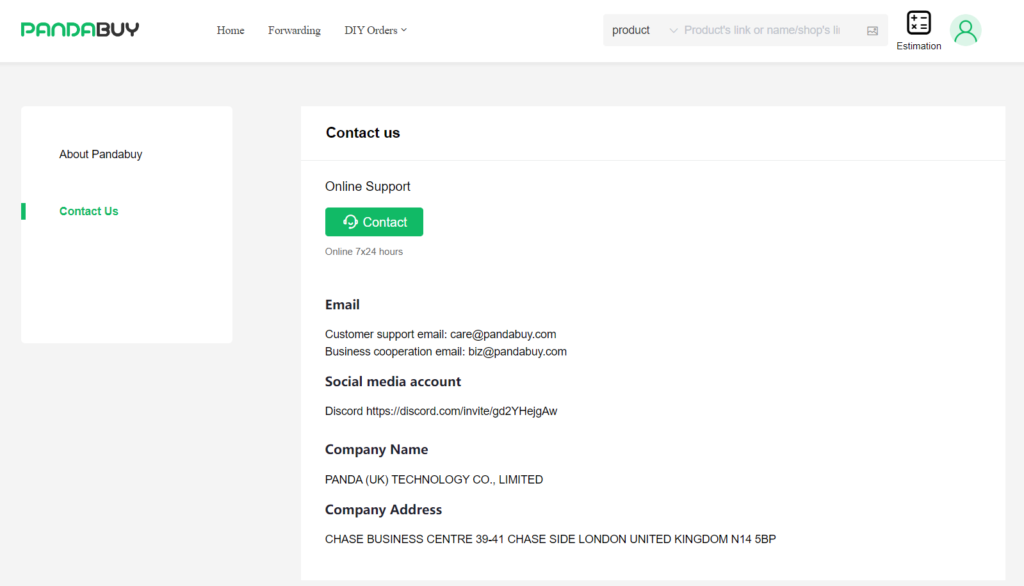A screenshot of the "Panda Buy" website is displayed, slightly wider than tall. 

**Top Section:**
- A white banner without borders.
- In the upper left corner, the logo reads "Panda Buy," with "Panda" in green text and "Buy" in black.
- To the right of the logo, a menu includes small text tabs: "Home," "Forwarding," and "Do-It-Yourself Orders," the latter featuring a drop-down button.
- Further right, a gray search box labeled "Product" allows the user to type queries.
- Adjacent to the search box, an "Estimation" button is visible.
- On the far right, a green person-like icon indicates a login option.

**Main Section:**
- The background alternates between solid gray, black, light gray, and black horizontal stripes.
- Near the top right, within a white box, "About Panda Buy" appears on one line, with "Contact Us" below it. "Contact Us" is highlighted in green with a corresponding green side indicator.
- To the right of this, a larger white box contains more details about the "Contact Us" section. The heading "Contact Us" is in bold, followed by a gray line.
- Below the heading, "Online Support" is listed with a green contact button featuring an icon, and an annotation reading "Online 7 times 24 hours."
- Below the online support section, various email support options are mentioned.
- Further down, a social media account section lists a Discord address.
- At the bottom, the company's name and physical address are stated.